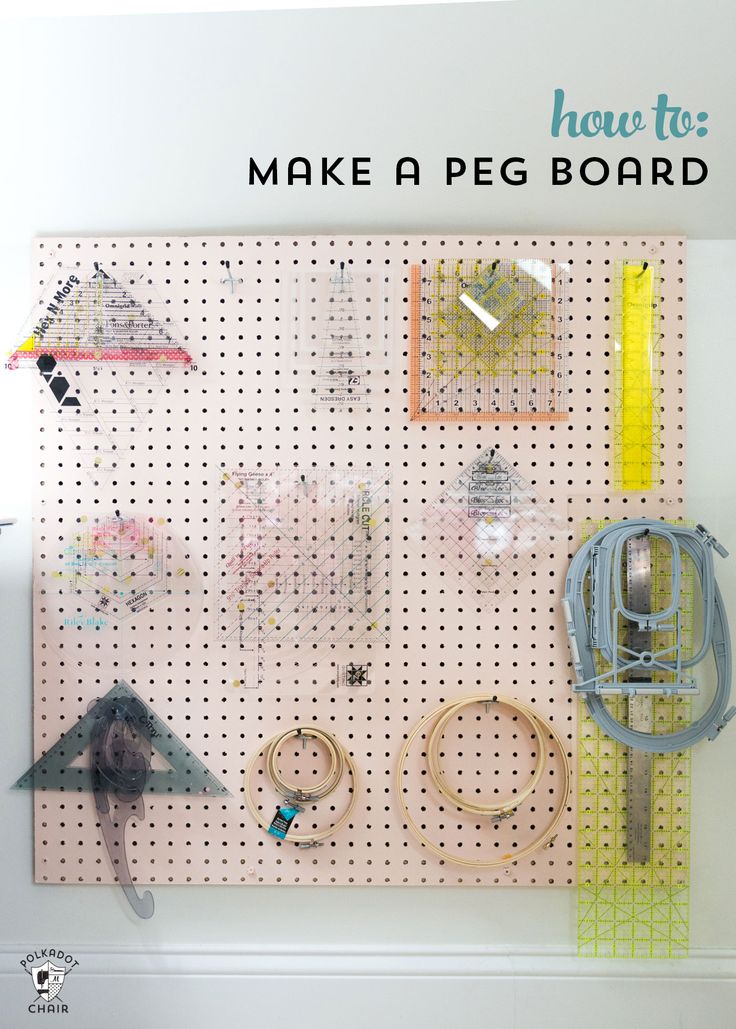This image displays a detailed instruction guide on creating a pegboard, resembling a Pinterest-style DIY project. The guide, set against a completely white background, features the title "How to" in a vibrant blue or teal color, followed by "Make a Pegboard" in black text. The pegboard itself, occupying the central portion of the image, appears to be a light peachy or light brown color, potentially influenced by the lighting. Various clear stencils and tools hang from the pegboard, some with red and black details, and others in yellow. Notable items include different ring shapes for additional projects. The pegboard hooks appear to be either black or silver with black tips. In the bottom left corner, there is a small icon featuring the words "Polka Dot Chair" alongside a black and white shield emblem.